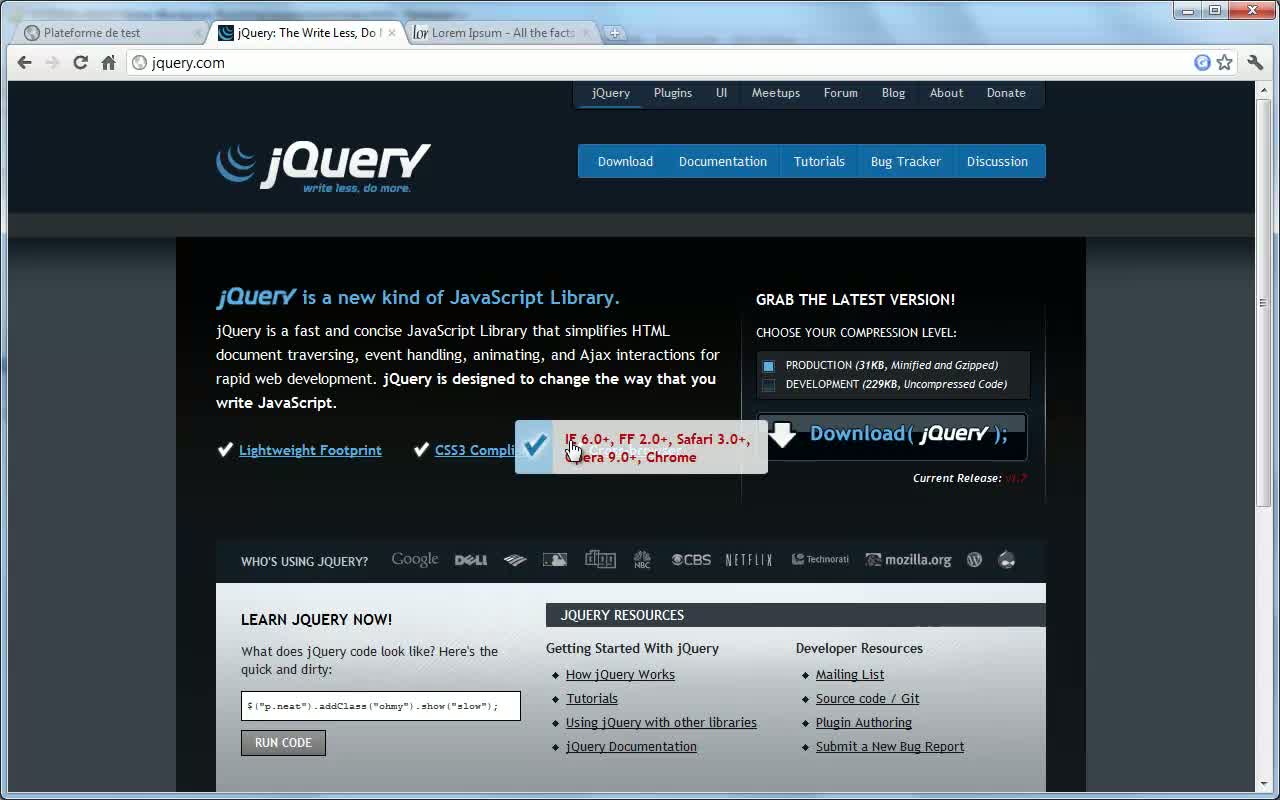The image displays a web page dedicated to jQuery, a renowned JavaScript library. At the top center, the jQuery logo is prominently displayed alongside its slogan, "Write Less, Do More.” Beneath this, jQuery is described as a "fast, concise JavaScript library that simplifies HTML document traversal, event handling, and animation.”

The right section features a download button accompanied by options for different compression levels for both production and development environments. Below this, a section provides various resources including tutorials, documentation, and a code example with an accompanying "Run Code" button.

The page is presented in a dark theme with red and white text, providing a visually striking contrast. At the very top of the browser window, there are other tabs visible, which appear to be unrelated to the current image. Positioned in the middle of the screen, the cursor highlights text specifications for browser compatibility, including "IE 6.0+", "FF 2.0+", and "Safari 3+", indicating the supported browsers at that time.